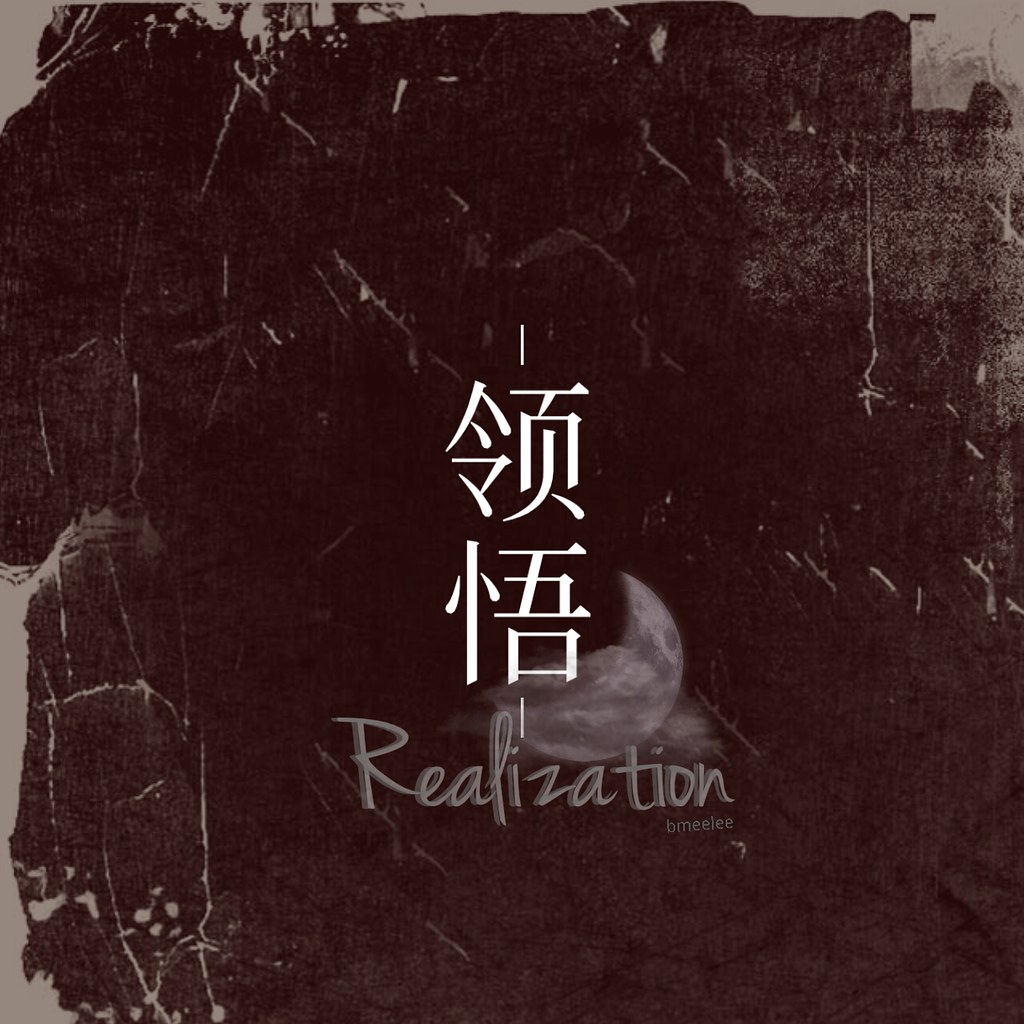The image features a prominently black, textured square background that appears aged and faded, with gray splotches and white scratches giving it a vintage feel. White squiggles, reminiscent of creases or cracks on weathered paper, are scattered throughout the surface. In the center of the square, there are two vertically stacked characters that appear to be Japanese or Chinese, followed by a depiction of a half moon. Below these elements, in a cursive gray font, the word "realization" is inscribed. Underneath "realization," in smaller, more subtle text, the characters "B-M-E-E-L-E-E" can be discerned, possibly indicating a name or title. The overall effect is an aesthetically distressed black-and-white composition, evoking a sense of timelessness and depth, perhaps suggestive of a vintage album cover.